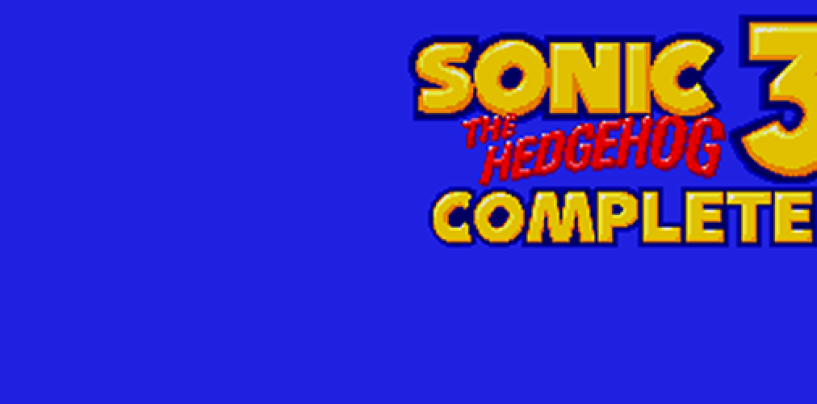This image is a detailed color graphic with a typography focus, set in a landscape orientation. It features a vivid blue background that dominates the entire image, with specific text elements positioned in the upper right corner. The text, styled in a mix of bright yellow, red, and other colors with dark tints and shadows, prominently reads "Sonic the Hedgehog 3 Complete." The title "Sonic" appears in large yellow letters, followed by "The Hedgehog" in smaller red letters with a smoke-style arc beneath it, and the word "Complete" in large yellow letters underneath. The entire title is outlined in black with a slight drop shadow, giving it a dynamic and three-dimensional appearance. The left half of the image remains blank, contributing to the overall clean and graphic design, reminiscent of an old video game title screen or a website banner.